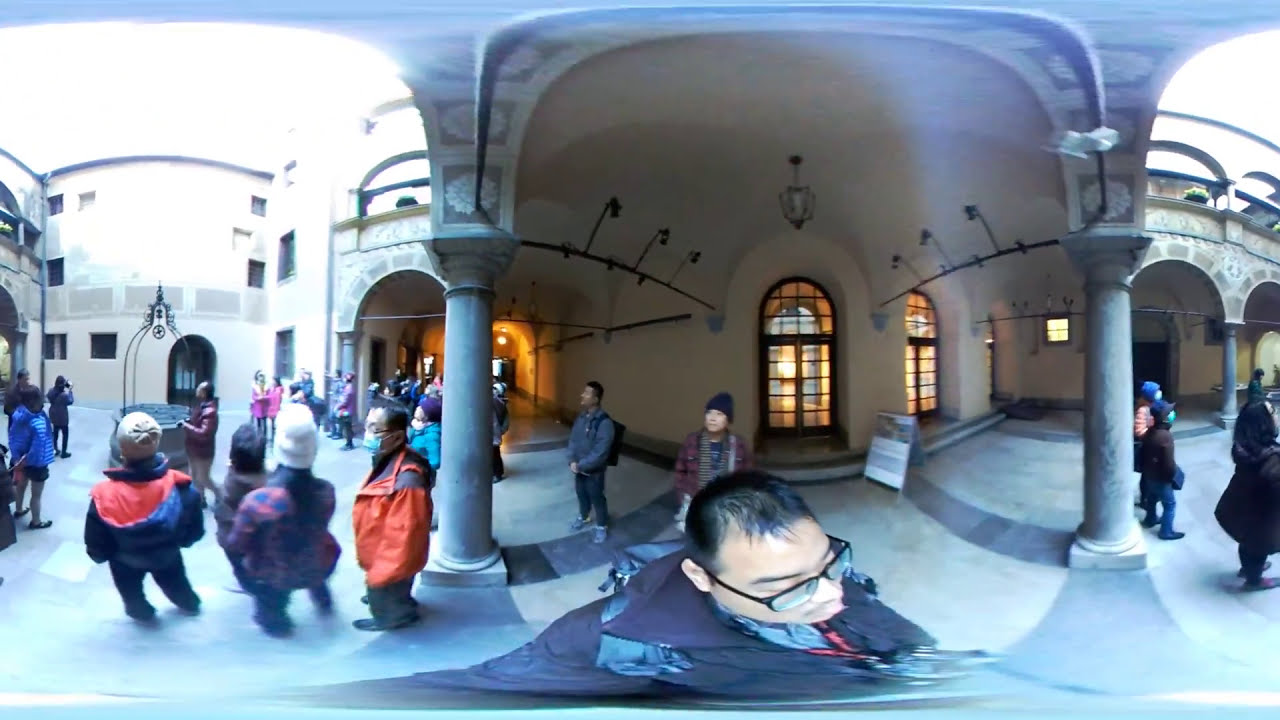The image depicts an exterior scene of a massive, historic building with a white facade, likely situated in an Asian location frequented by tourists. The building features old-style architecture with stone-colored walls, archways, and pillars, creating an imposing and visually striking structure. The central focus of the image highlights a man with black-rimmed glasses, wearing a jacket, and holding a selfie stick to capture a widescreen shot. He stands amidst a crowd of people, most of whom are clad in coats and beanies, indicating cold weather. Several individuals wear masks, reflective of contemporary health precautions.

In the middle-left area of the image, there is a well around which tourists gather, some taking pictures and many looking upward, possibly at an architectural detail or an attraction above. The right side of the image also shows a group of people, many of whom are masked and dressed in jackets and jeans, similarly captivated by something above. The background reveals large, illuminated double doors surrounded by the interior structure, contributing to the ambiance with warm light filtering through glass panes. A sign near the doors suggests this building is a significant historical or cultural site, offering information to the visitors.